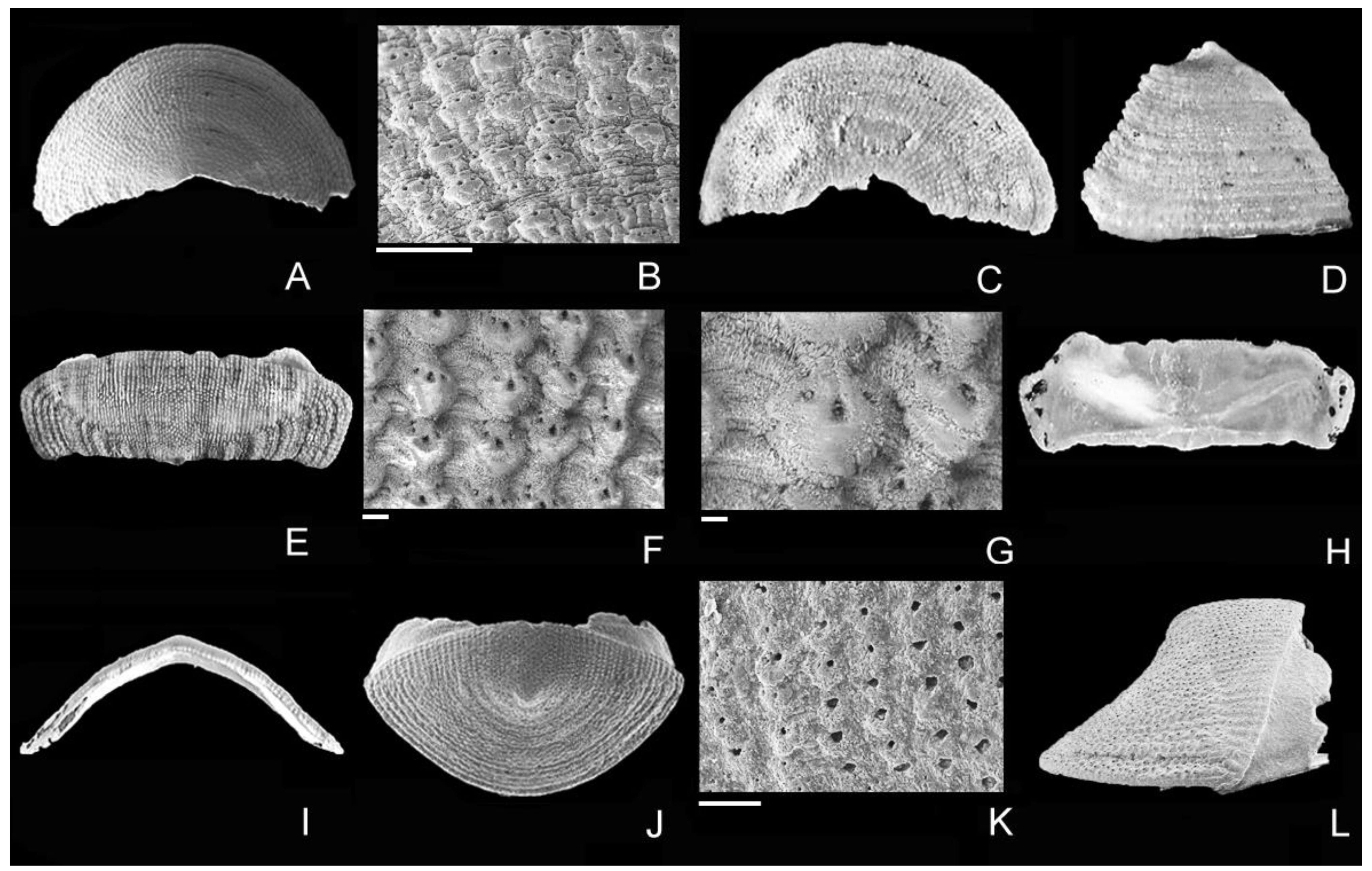The image displays 12 grayscale photographs labeled A through L, set against a black background. Each photograph captures a detailed close-up, possibly of microscopic subjects or small natural objects, presenting an array of intriguing textures and patterns. Photographs A, C, and J depict rounded shapes featuring radiating lines from a central point, resembling concentric rings often found in tree trunks or shells. Images B, F, G, and K showcase dot details or scale-like patterns, suggestive of textured surfaces like bumpy rocks or microscopic structures. Photograph I presents an object that appears to be a curved bone or a stick, while L features an element reminiscent of a shark's tooth or possibly a fossilized shell. The collection appears to serve a scientific purpose, perhaps as a reference for documenting various natural or biological textures and shapes.